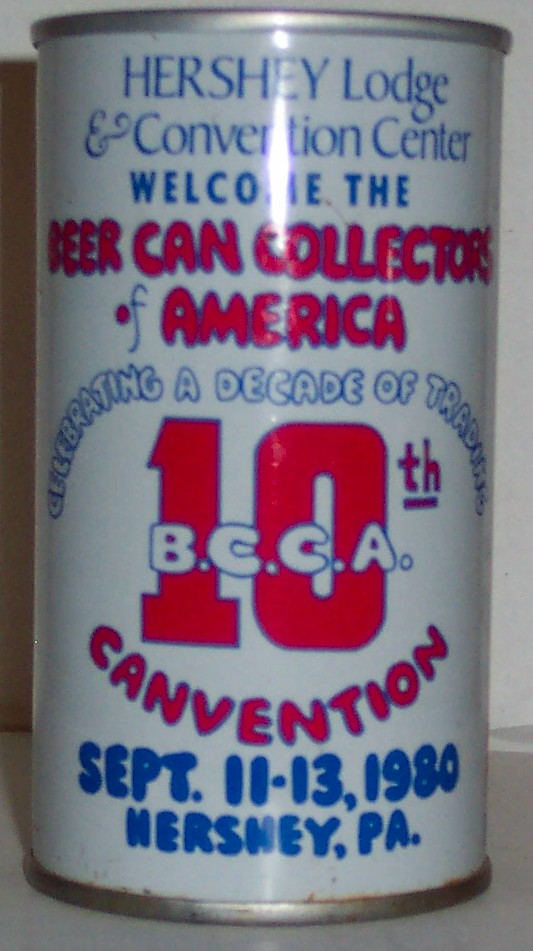This photograph showcases a collectible beer can that prominently features a variety of colors and text. The can has a primary background of white, with notable lettering in blue, pink, and white fonts. At the top, the blue text reads, "Hershey Lodge and Convention Center. Welcome the," followed by the pink text proclaiming, "Beer Can Collectors of America." In white text, it continues with, "Celebrating a Decade of Traditions," accompanied by the number "10th" in pink. The abbreviations "B.C.C.A." appear in white, with "Canvention" in pink. Further down, blue text specifies the event dates and location: "September 11th to 13th, 1980, Hershey, Pennsylvania."

The can is finished with silver rims at both the top and bottom edges. The white surface of the can displays some rust spots, particularly noticeable at the top and bottom. These signs of aging add character to this vintage collectible item.